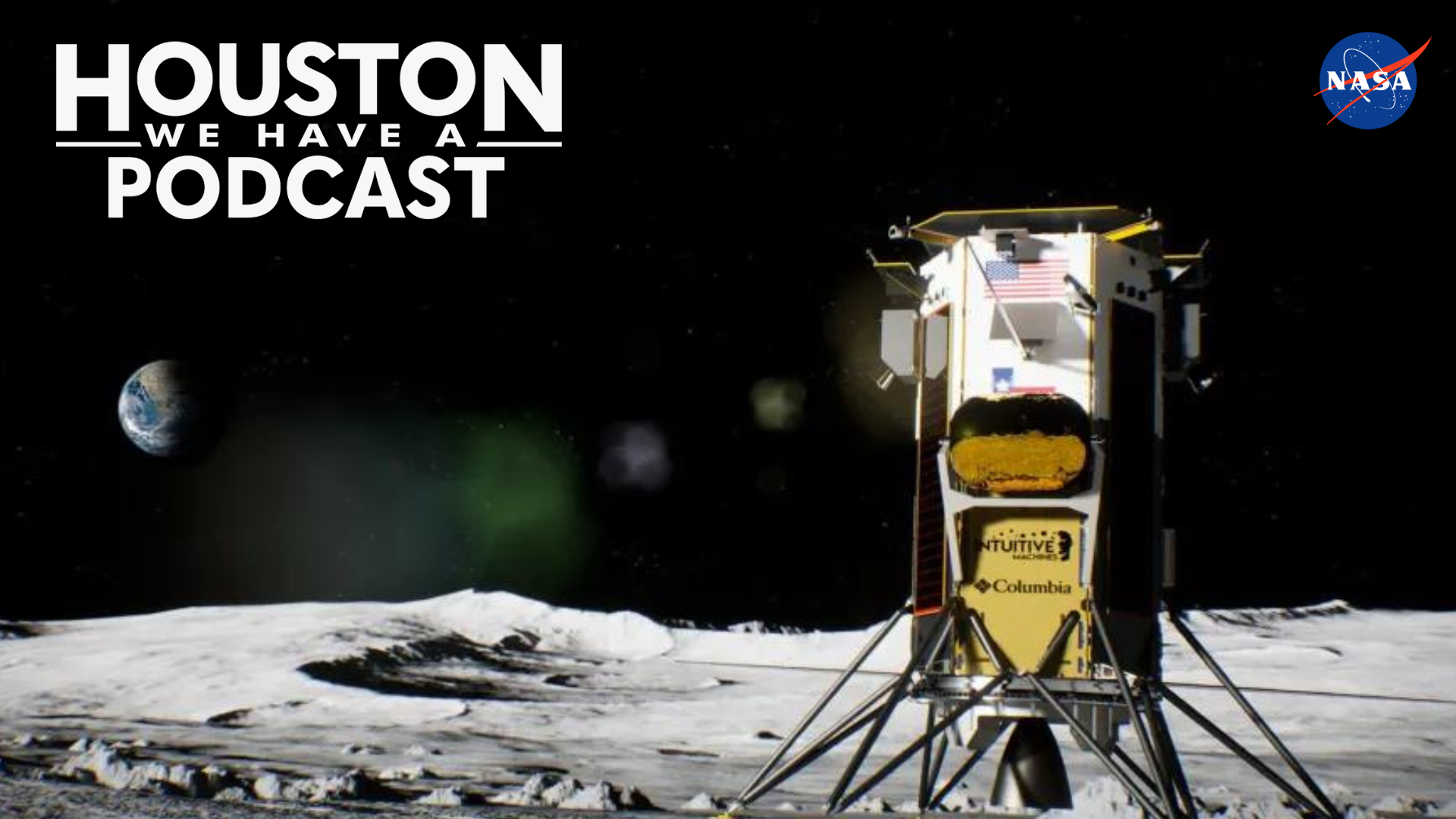This image is an advertisement for a podcast, featuring a full-color photograph of a spacecraft on the moon, evocative of the lunar lander from the 1960s. The lunar surface is gray and craggy, occupying the bottom portion of the image. Above this, the horizon stretches into the black emptiness of space, where a small image of Earth appears to the left. In the upper left corner, white text reads "Houston, we have a podcast," with unique formatting, using two dashes for emphasis. The upper right corner displays the iconic NASA logo, a blue circle with the word "NASA" in white and a red forked vector crossing it. Dominating the moon’s surface is the lunar module, labeled "Columbia," featuring an American flag and details in black and gold. The overall composition highlights the stark contrast between the lunar landscape and the vastness of space, blending historical elements with modern promotional visuals.